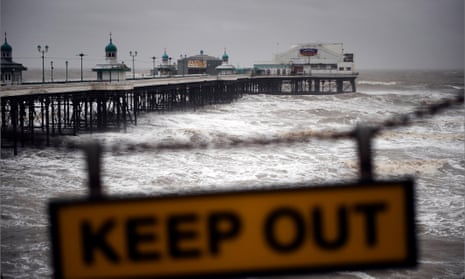A blurred orange and black "Keep Out" sign hangs from a black chain in the foreground of the image. Beyond the sign, a long pier extends out into a tumultuous, frothy ocean under a stormy, gray sky. The water is rough and choppy, with visible white foam and brownish hues underneath. The pier, elevated above the water, leads to two large buildings at its end, possibly restaurants or a combination of a restaurant and a fishing area. Light poles are spaced along the pier, contributing to its industrial appearance. In the distance, another building on a separate pier is visible to the left, with some trees faintly seen in the background.